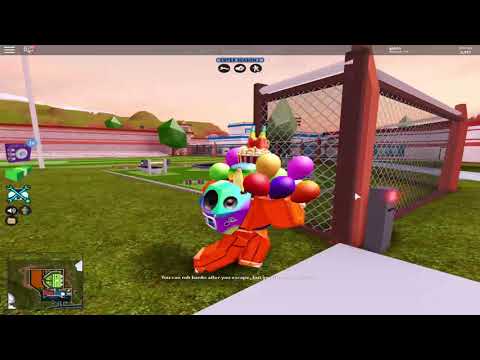In this detailed screenshot from a third-person video game, we see a blocky, orange-colored character standing approximately five feet away from the camera in a vibrant grassy field. The character, adorned with a teal and purple backpack featuring black speakers, has their head obscured by a cluster of colorful balloons in various hues—yellow, purple, green, red, gold, pink, and orange. To the left of the character is a short, wide building with white walls trimmed in red, and to the right, they stand in front of a rectangular fence enclosure made from wooden poles topped with a silver chain link fence. Surrounding the grassy area are blocky trees with flat sides and pointy tops. In the lower left-hand corner of the image, a small mini-map and directional key are visible, providing gameplay instructions and the character's position within the field.